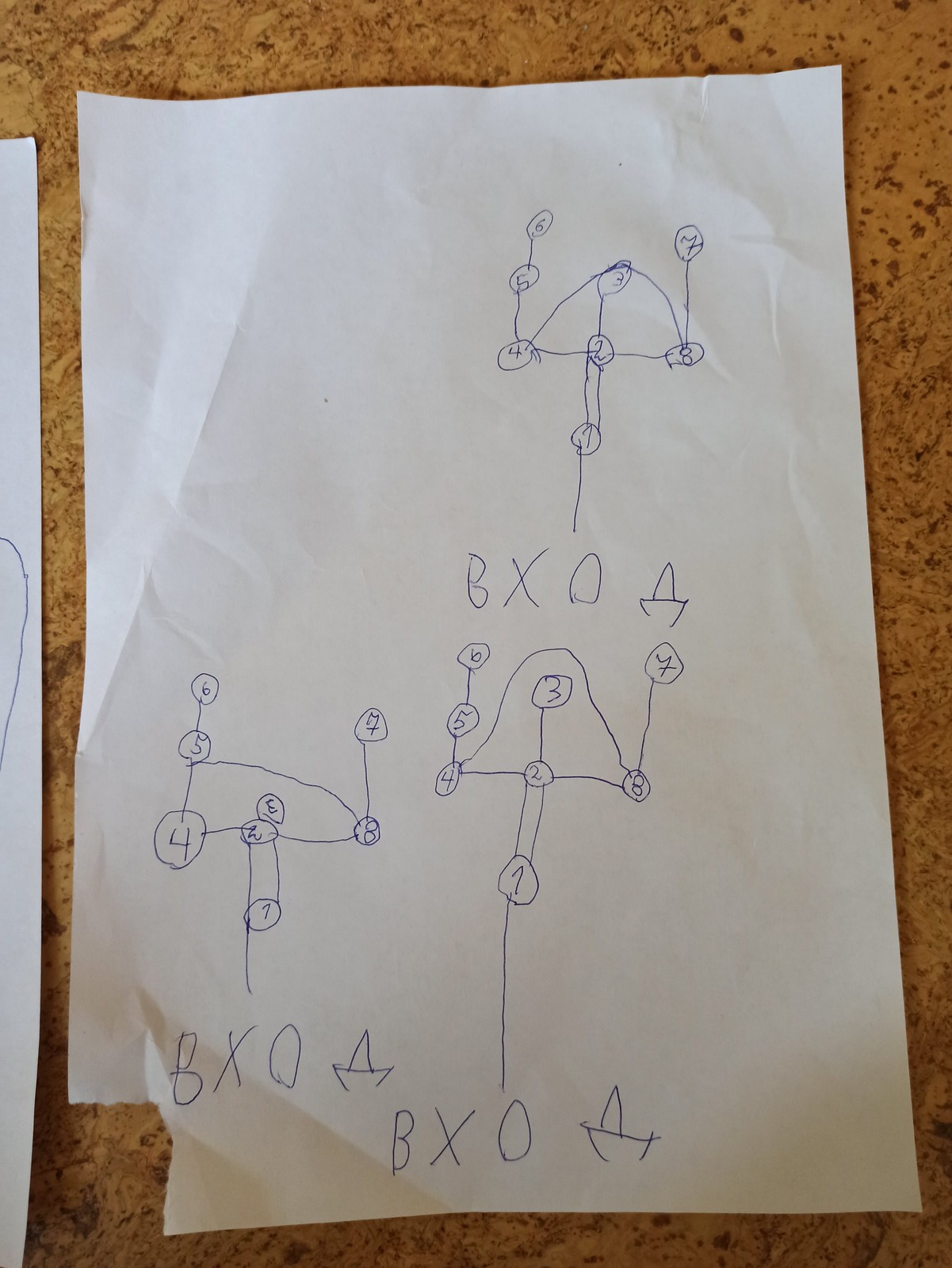The image features a predominantly yellow and brown background speckled with dark spots scattered throughout. At the center, there is a white sheet of paper adorned with intricate blue ink drawings. On this paper, the bottom left corner is marked with the letters "BXO," which also appears at the very bottom and heads upward.

To the left of these letters, a series of connecting lines and circles are illustrated. In the top left corner, the numbers 6 and 7 are marked, with 6 linked to a 5th circle, which descends to a 4th circle, then extends over to a 3rd and 2nd circle. The bottom includes a 1st circle, situated with an 8th circle on the right, leading back up to the 7th circle. Further to the right, additional circles and archways are interconnected by lines. The sequence follows a path from a 1st circle, progressing through a 2nd and 3rd circle, then looping back down to the 2, ascending to the left through circles 4, 5, and 6, descending again through 5 and 4, moving right to 2, extending to 8, and finally ascending to 7.

Above the entire arrangement, "BXO" is inscribed again. Above this, there is a distinctive drawing resembling a small boat or bowl with tiny triangles protruding from it. Above this drawing, there's a recurring pattern of circles numbered 1 through 8, connected by various archways and lines, showcasing a complex and detailed diagrammatic structure.